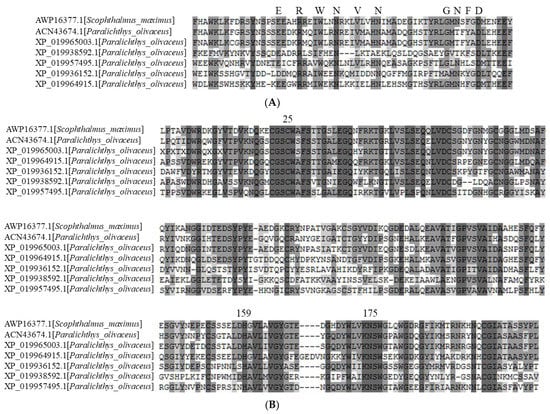This is an image resembling a printer ink test, showcasing four distinct sections, each filled with various letters and numbers. The sections, structured in blocks, manifest in a black and white palette accentuated with grayscale variations, including gray, silver, and darker tones, indicative of different ink densities. The first section, labeled 'A' at its bottom, and the fourth section labeled 'B' at its base, are particularly insightful: the intervening sections feature numbers such as "25", "159", and "175". Each block contains eight rows of sequences of seemingly arbitrary letters and numbers, creating a chaotic text appearance. Codes such as "XP019938592" and "AWP16377.1" are visible amidst the jumble. Random sequences, like "YQQDYLV" and "ERWNN", mixed with sporadic configurations like "GNSU", suggest a lack of coherent words, imparting a sense of gibberish. The sections also exhibit inconsistent levels of ink coverage, with upper sections appearing less disrupted compared to the heavily smudged or splotched bottom segment, evoking thoughts of a printer malfunction.